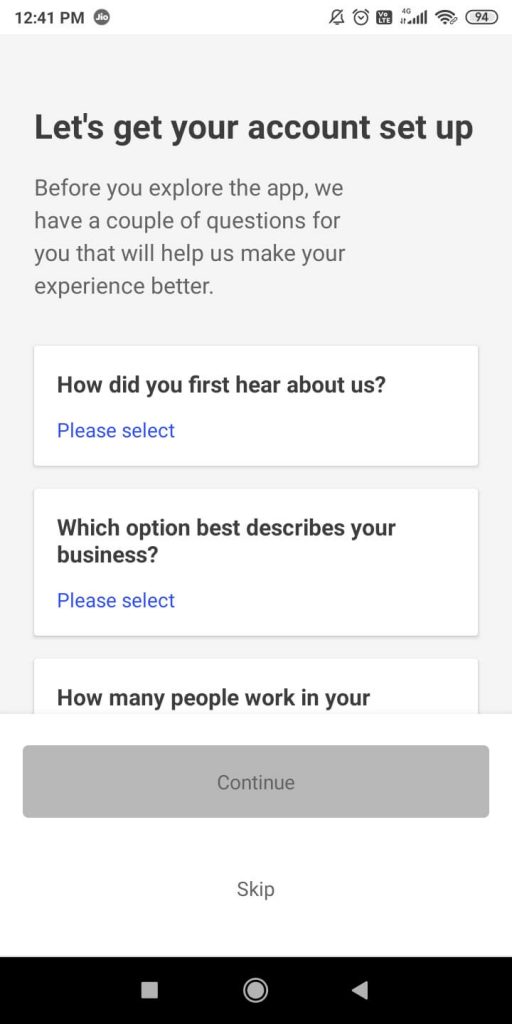The image depicts a cell phone screen displaying the setup process of a business-related app. At the top, the time reads 12:41 p.m. The right corner shows an icon for notifications, which have been turned off, along with indicators for an active alarm, 4G connectivity, cellular signal strength, Wi-Fi, and a battery level at 94%. 

Below the status bar, a message invites the user to set up their account with the prompt, "Before you explore the app, we have a couple of questions for you that will help us make your experience better." The first question asks, "How did you first learn about us?" followed by a blue text option to "Please select." The next question inquires, "Which option best describes your business?" also followed by a blue text option to "Please select." Another question begins with "How many people work in your..." but is cut off and incomplete.

At the bottom of this setup page, there is a gray "Continue" button, and beneath it, a gray "Skip" button. The phone’s navigation bar appears as a black strip containing a white square for the home button, a circle, and a left arrow for back navigation. The overall color scheme of the interface includes shades of black, white, gray, and blue. There is no clear indication of the app's identity or the specifics of the account being set up, but the context clues suggest it is tailored towards business users.